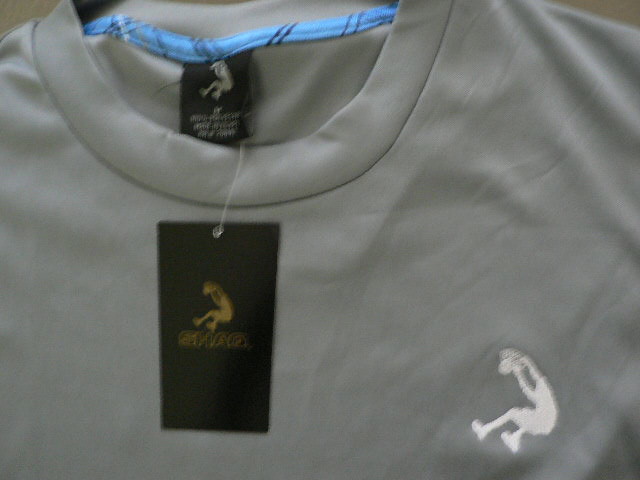This photograph, taken in dim lighting, shows an extreme close-up of the top portion of a gray athletic t-shirt, primarily focusing on the collar and upper chest area. The t-shirt features a blue stripe along the inside back of the neck. At the top of the shirt, a black label with a white Shaq logo is sewn inside the neck hole. Below this, a black hang tag with a gold version of the same logo—including an image of a person hanging from a basketball hoop and the text "Shaq"—is attached. Additionally, the same white Shaq logo is embroidered on the lower right corner of the shirt. The fabric appears slightly wrinkled on the right side, and the image's dim lighting makes it challenging to discern the exact shade of gray.